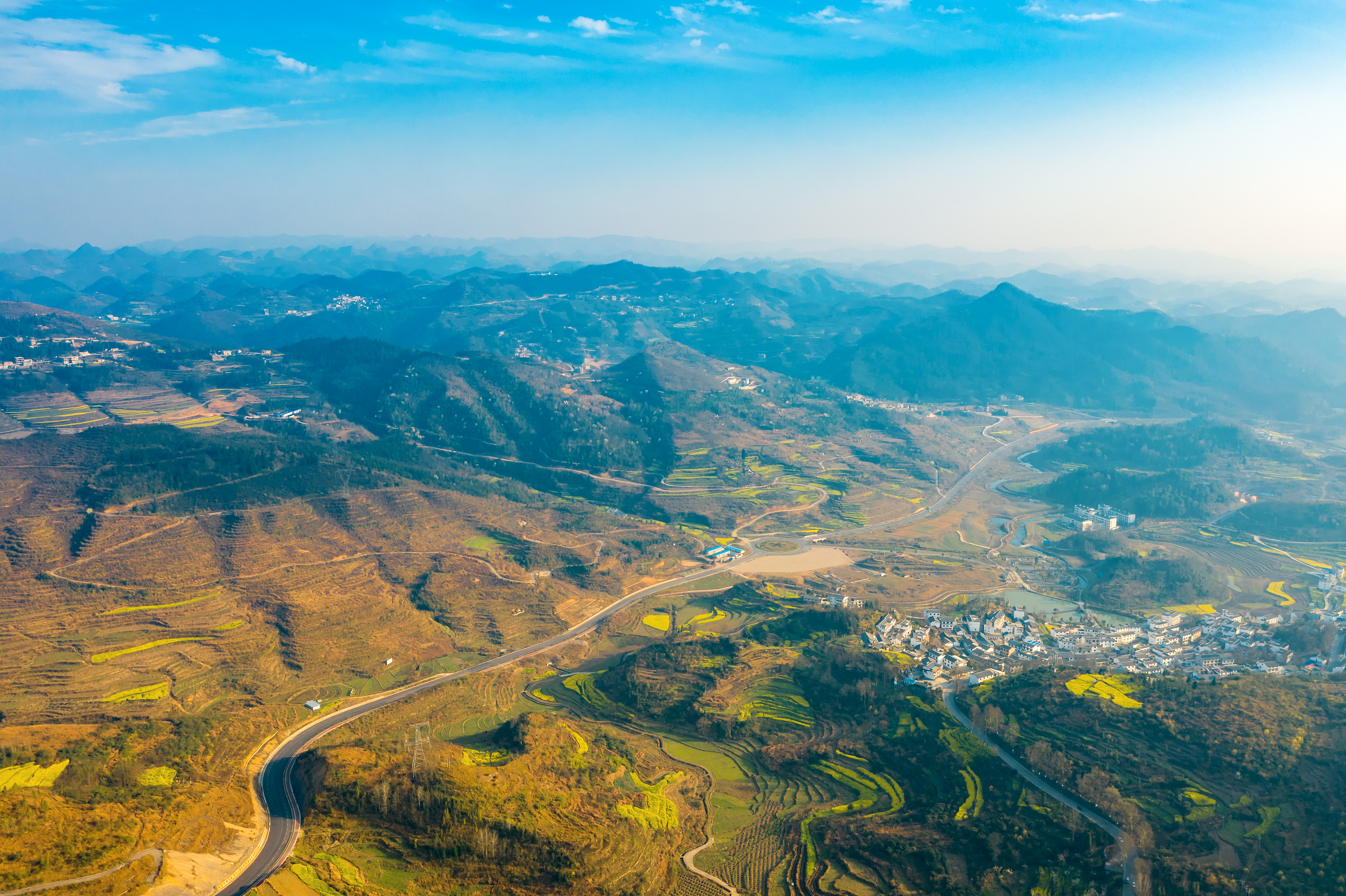This is an expansive aerial photograph showcasing a vibrant landscape, divided into a top third sky and a bottom two-thirds terrain. The sky is a mix of white and gray hues with scattered clouds. The foreground prominently features a vivid patchwork of green and gray fields laid out in terraced layers across the rolling hills and mountains. These terraces, resembling stairs, are interspersed with snaking roads that traverse the mountainous terrain. On the right side of the image, there is a smaller city with numerous white buildings surrounded by verdant fields and bodies of water nestled into the mountain slopes. To the left, more mountains dominate the view, characterized by brown and green hues. The distant background fades into light blue mountains, providing a fuzzy, ethereal quality due to the vast distance. This bird's eye view captures the intricate balance between nature and human habitation, highlighting fields, residential areas, and a network of roads that blend seamlessly into the breathtaking landscape.